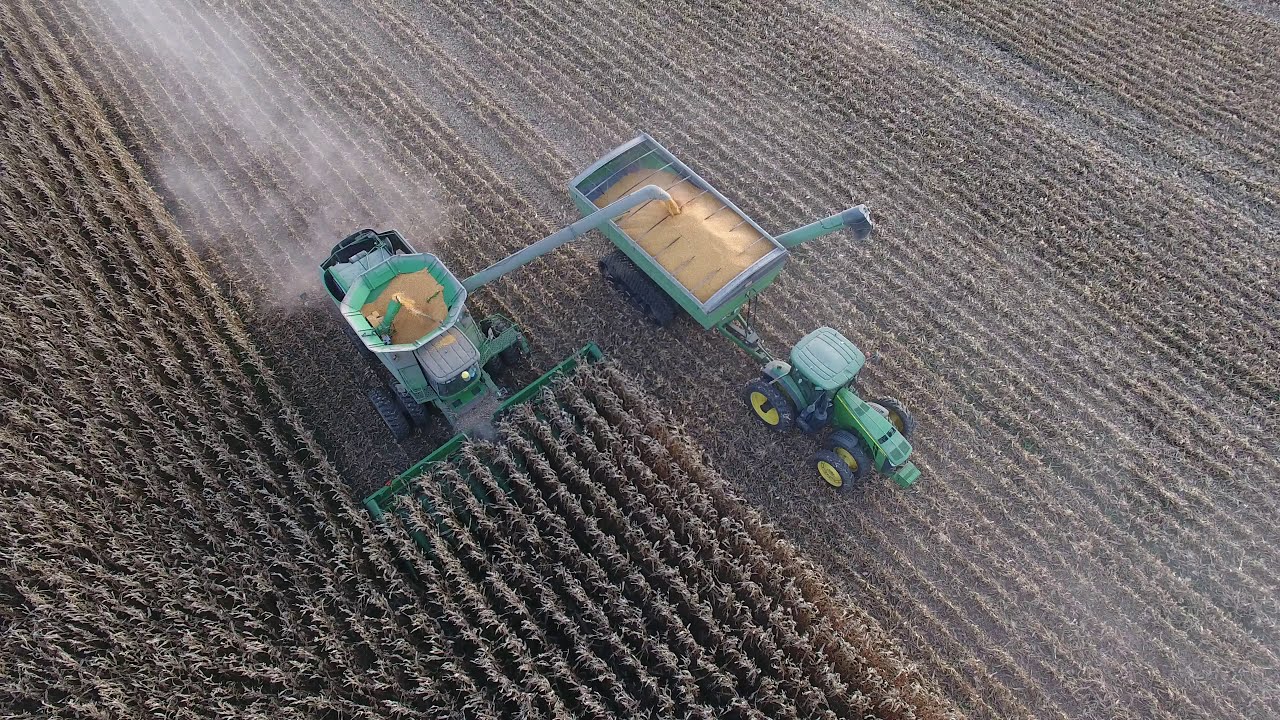This detailed aerial photograph, captured by a drone, shows an expansive wheat field during harvest. The landscape-oriented image features two green John Deere vehicles with yellow wheels operating in tandem. A thresher on the left, driving in a diagonal direction, is actively chopping down rows of tall, golden wheat and channeling the grain through a cylindrical tube into a rectangular container towed by a tractor on the right. The thresher's path, marked by distinct lines angled at 45 degrees counterclockwise, shows the already cultivated areas of the field which appear tan against the uncut wheat. The container being towed by the tractor is nearly full, while the thresher continues to harvest and fill it with grain. Both vehicles cut through the standing wheat, demonstrating the coordinated effort in the agricultural process.